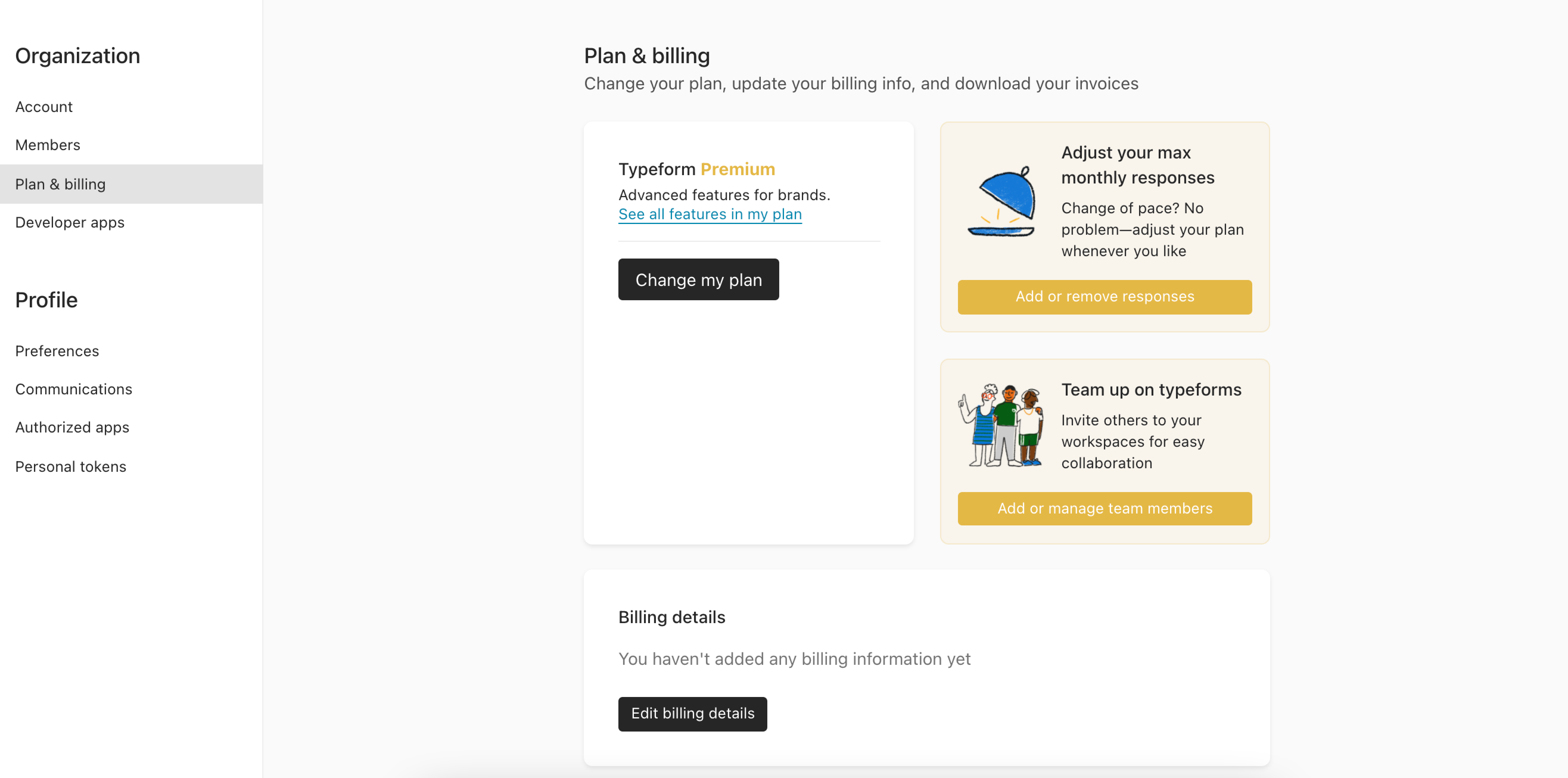Sure, here is a detailed and cleaned-up description of the image:

---

In the image, there is a side menu positioned on the left, formatted as a list for navigation. The items from top to bottom are: 

1. **Organization**
2. **Account**
3. **Members**
4. **Plan and Billing** (highlighted in grey)
5. **Developer Apps**

Below the "Developer Apps" section, there is a "Profile" section with the following sub-items:

1. **Preferences**
2. **Communication**
3. **Authorized Apps**
4. **Personal Tokens**

The text within this side menu is written in black, and the background is white.

To the right, in the main content area which is centered, the page begins with the header "Plan and Billing". This section provides the functions to "Change your plan, update your billing info, and download your invoices." 

Below this header, it indicates that the user is on a "Typeform Premium" plan, where "Premium" is written in orange and "Typeform" in black. Beneath this, there is a description in black text that reads "Advanced features for brands", followed by a clickable link in blue that says "See all features in my plan." Additionally, there's a black button with white text that says "Change my plan."

On the right side of the main content, there are two sections. The upper section provides an option to "Adjust your max monthly responses. Change of pace? No problem, adjust your plan whenever you like." Next to this option is a blue icon, and an orange button below it that says "Add or remove responses." The text background here is light orange.

The lower section on the left highlights "Team up on Typeforms." It encourages users to "Invite others to your workspace for easy collaboration." This is followed by another orange button that says "Add or manage team members", accompanied by an icon of team members.

At the bottom of the main content area is a "Billing Details" section. It informs the user with the note, "We haven't added any billing information yet," followed by a black button with white text that reads "Edit billing details."

---

I hope this thorough description aligns well with the image depicted.